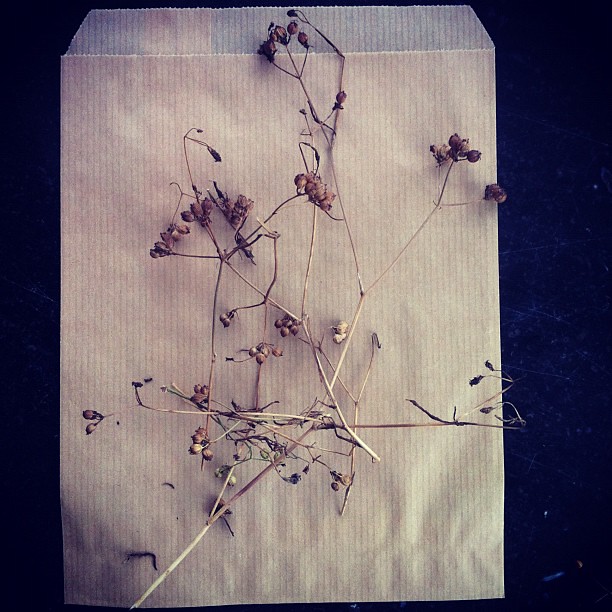In this photograph, delicate, dried plant stalks adorned with small, withered seed pods or flowers are scattered randomly across a light brown, clean piece of cardboard, which might be mistaken for a paper bag. The cardboard features visible vertical corrugations running from top to bottom. These fragile, brown plants highlight their dry, stick-like nature, further emphasizing their lifeless state. Resting atop a dark background, possibly blue or black, the overall scene is bathed in a subtle, rustic charm, with the dark hues of the background providing a stark contrast that accentuates the details of both the plants and the cardboard. The cardboard appears slightly bent towards the bottom left, casting soft shadows that add depth to the image. The entire composition is tinted in such a way that it mutes the true colors, giving the entire scene a monochromatic appearance that enhances its rustic and timeless ambiance.